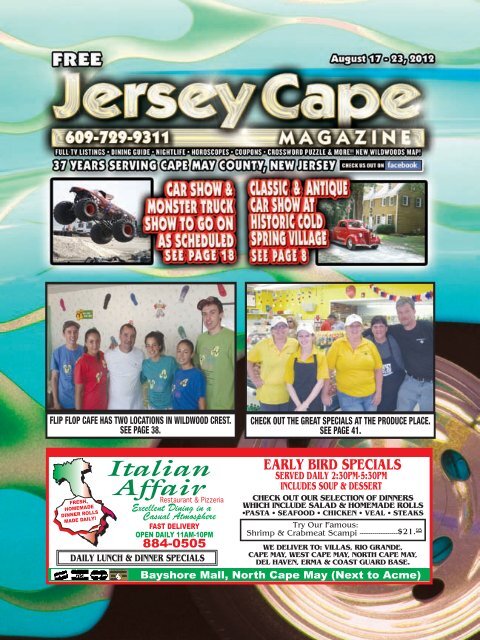The vibrant, colorful cover of the Jersey Cape Magazine, a free local circular paper, announces its weekly edition for August 17th through 23rd, 2012. The title, "Jersey Cape," is elegantly stylized with gold and light gold lines that shine in various sections. This edition marks 37 years of service in Cape May County, New Jersey. The background features a swirling green pattern painted onto a car tire and hubcap.

Central to the cover are four distinct, boxy photographs showcasing different local events. The top image captures an airborne monster truck, accompanied by text promoting a Car Show and Monster Truck Show with details available on page 18. Another image to the right depicts an old red sedan parked in front of a tall brick house, highlighting the Classic and Antique Car Show at Cold Spring Village, with more information on page 8. Further down, there's a lively group of employees in bright colorful t-shirts from the Flip-Flop Cafe, which has two locations in Wildwood Crest—additional details on page 38. Adjacent to this, a photograph features middle-aged and older people in mostly yellow shirts, some wearing aprons inside a grocery store, promoting great specials at the Produce Place, with further details on page 41.

Finally, at the bottom of the cover, there's a sponsor advertisement for Italian Affair Restaurant, detailing its specials and menu items, adding a delightful touch to this well-rounded community publication.